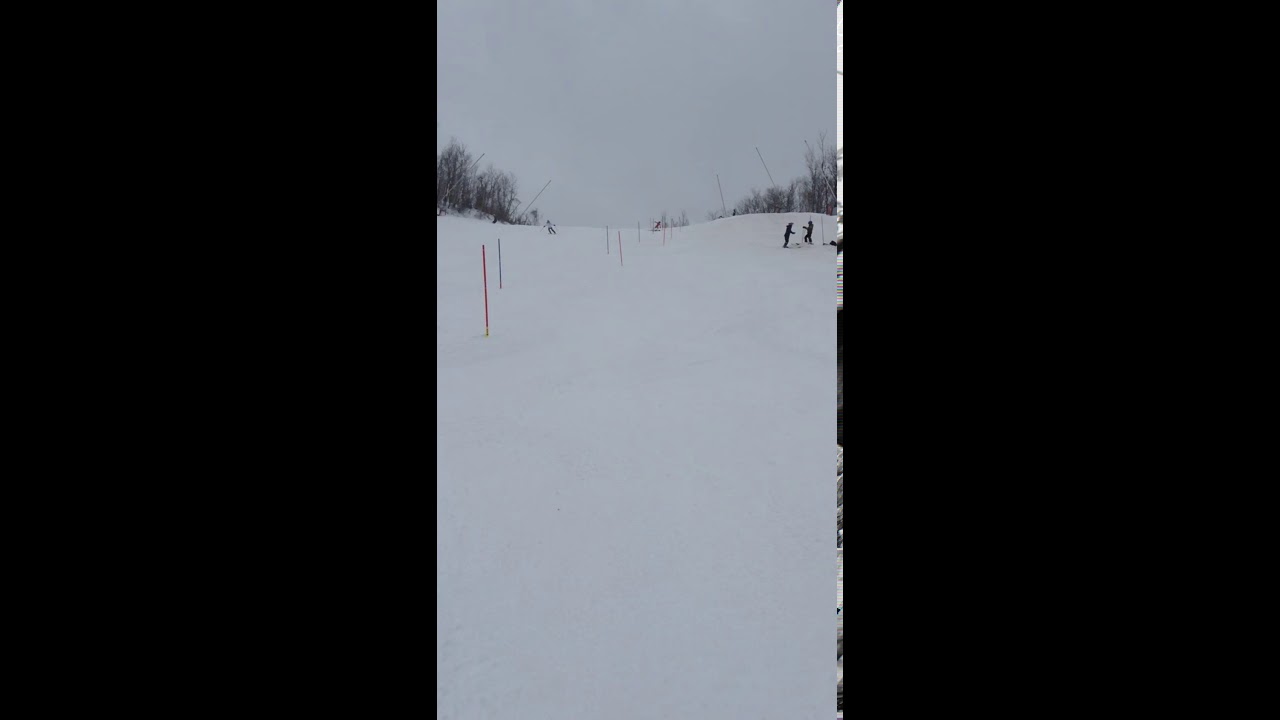A tall, vertically-oriented photograph captures a snowy ski slope, flanked on either side by thick black borders. The main section of the image is dominated by an overcast sky, blending into a completely snow-covered hill. The top of the hill, visible in the upper third of the image, is dotted with leafless dead trees and brownish bushes. Just below this horizon line, a small skier is making their way down the slope. On the far right, two barely visible individuals, dressed likely in black, appear to be standing still, possibly facing each other in conversation. Scattered along the slope are six to eight red poles, possibly marking an obstacle course for skiers to navigate. The sky remains overcast with no hint of sunlight, creating a bleak but serene winter scene.